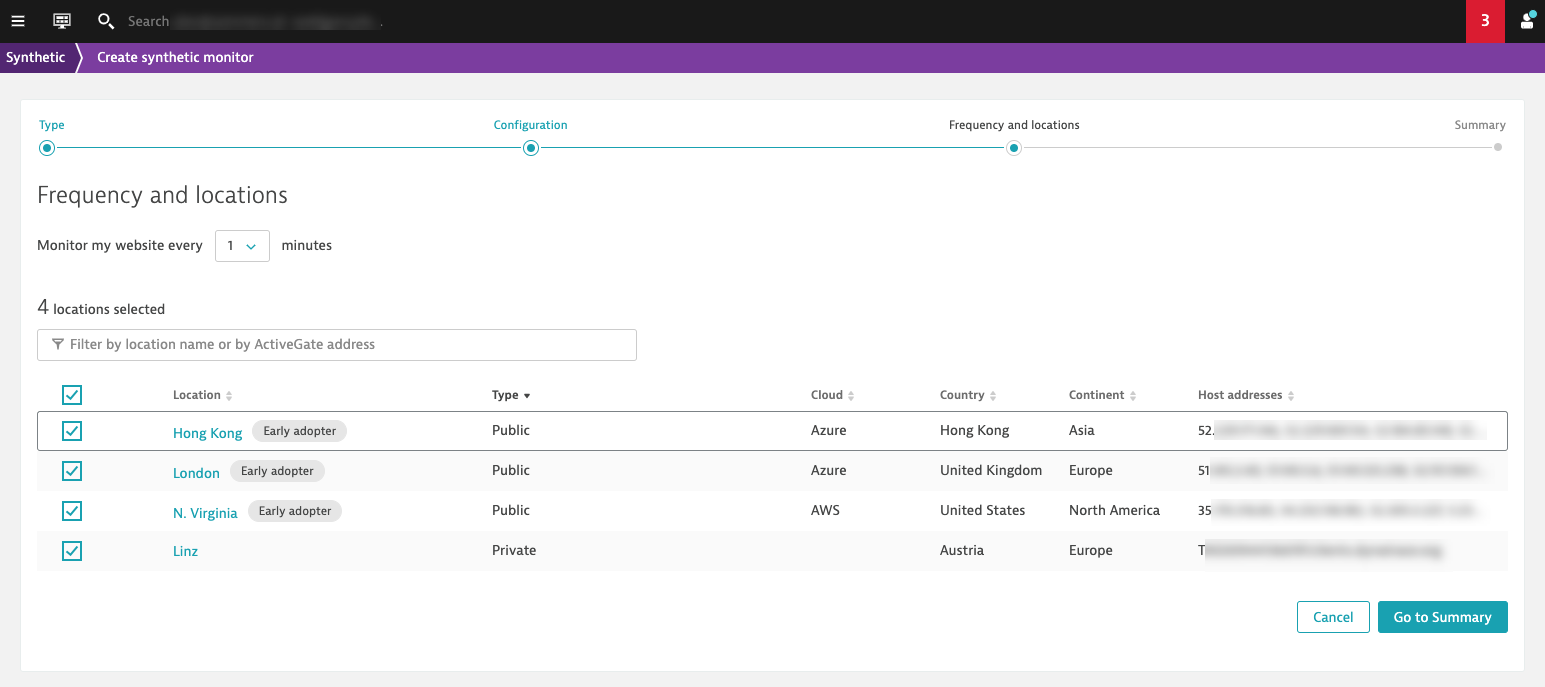A screenshot of a webpage used to create a synthetic monitor. At the top left, the page is titled "Create Synthetic Monitor." The main content features configurable settings for monitoring a website’s performance, including sections for "Frequency" and "Locations." The default monitoring frequency is set to every one minute, but this can be adjusted.

The page specifies that the monitoring uses four selected locations: Hong Kong, London, North Virginia, and LINZ. Hong Kong and London utilize Azure hosting services, North Virginia uses Amazon Web Services (AWS), and LINZ is a private server. 

A section below shows a status bar with columns labeled "Type," "Configuration," "Frequency and Locations," and "Summary." At the bottom right corner of the page is a "Go to Summary" button, stylized in a distinctive aqua or teal color. A search bar is positioned at the very top left of the page for easy navigation.